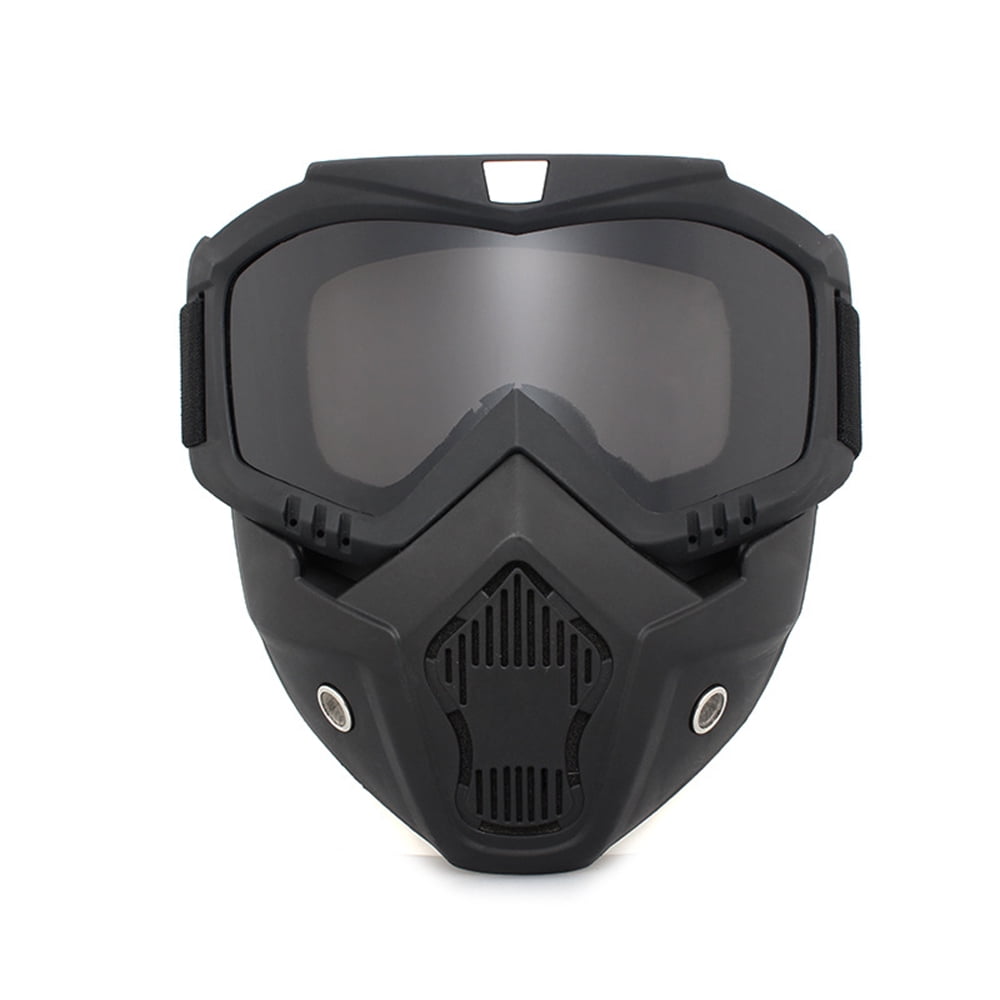This image depicts a tactical-style mask primarily used for activities such as paintball or potentially snowboarding. The mask is made of black plastic material and features a wide, slightly transparent visor at the top, designed to protect the eyes. The visor connects to a pair of goggles with a black, elastic strap securing it on the wearer’s head. Below the goggles, the front of the mask tapers down to a triangular shape, which snugly fits the contours of the face. This section of the mask includes multiple slots and pentagon-shaped cuts designed for ventilation, allowing the user to breathe easily. Additionally, there are two silver or white circular components on the lower left and right sides of the mask, which may serve as additional vents or attachment points for filters. Overall, the mask is notably wider at the top, where the goggles are, and gradually narrows down towards the chin, providing comprehensive facial coverage.